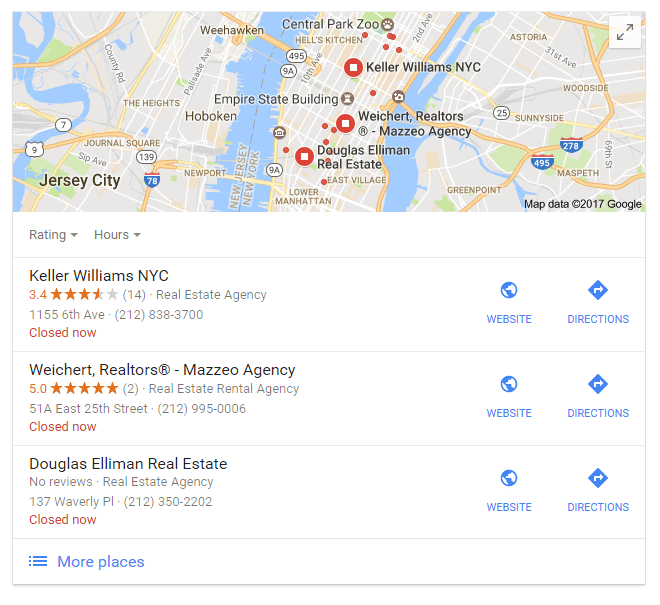In this image, we see a screenshot of a Google search result featuring a map centered around Jersey City and the Empire State Building. The map is adorned with red markers indicating various real estate agencies. Below the map, there's a detailed list of three highlighted locations:

1. **Keller Williams NYC** - Rated 3.4 stars based on 14 reviews, marked as closed.
2. **White Shirt Realtors from Mazo Agency** - Rated 5 stars based on 2 reviews, marked as closed.
3. **Douglas Elliman Real Estate** - No reviews, marked as closed.

Each location on the list features a "Website" button on the left side and a "Directions" button on the right side, offering the user quick access to further information and navigation options.